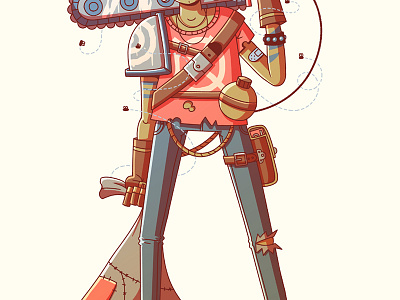This image depicts a stylized cartoon character, capturing only a partial view from the top of the chin down to above the ankles. The character, assumed to be a man, wears various garments and accessories suggestive of a rugged, possibly post-apocalyptic environment. His attire includes blue jeans with a notable tear at the knee exposing some skin, and a tattered orange or salmon t-shirt with a white circle and cross design. His hands are clad in brown gauntlet gloves, and he holds a patched knapsack in one hand. Around his waist, there’s a belt supporting a circular device, perhaps a canteen, along with additional ropes. A holster with a gun is strapped to his upper left thigh, and on his right leg, there is an indistinct brown item. He also sports a shoulder pad on his right side. His left arm is bandaged and adorned with a black studded bracelet featuring blue dots. A winged contraption, the specifics of which are unclear, is affixed to his back, adding to the complexity of his appearance. The character also has a possible machete and what looks like a chainsaw behind his head. Flies buzz around him, enhancing the sense of desolation and grime in the scene. The image cuts off at the top and bottom, leaving the face and lower legs out of sight.